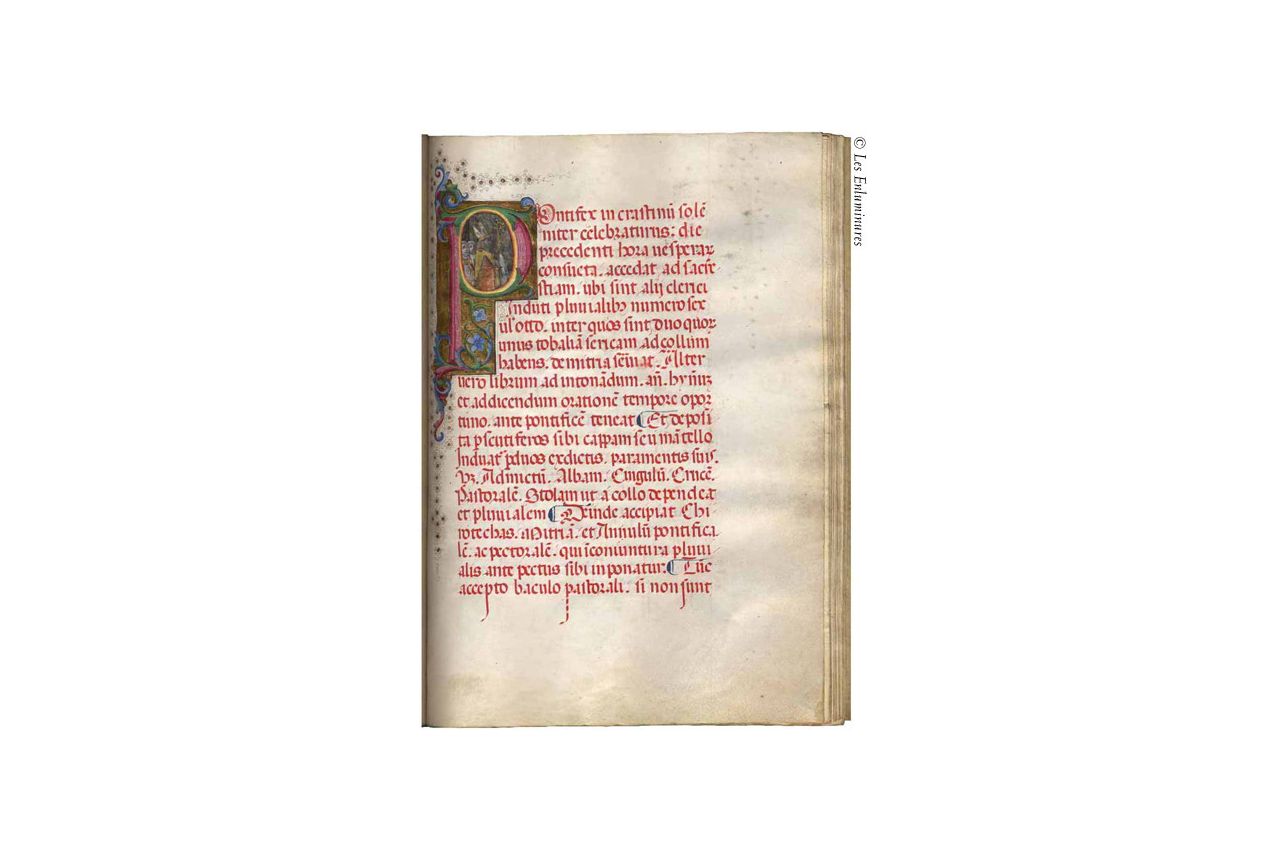The image depicts a single, aged page from an old book or pamphlet, distinguished by its worn and crinkled pages that fade from white to light brown. The binding on the left is brown and no book cover is visible. The page is filled with text in red font, which appears to be in a foreign language—possibly French, as indicated by the partial phrase "Les Enlilamerentes" on the upper right of the page. The text, resembling Latin cursive, is neatly arranged in multiple rows. To the left of the text is an illustration of a man with long hair, adorned with a crown and dressed in a red robe. Below this illustration are a couple of blue flowers positioned to the left of where the text starts. Additionally, there is a decorative element—an ornate circular initial, likely starting with the letter "P", encapsulating a small image with dot embellishments around it.